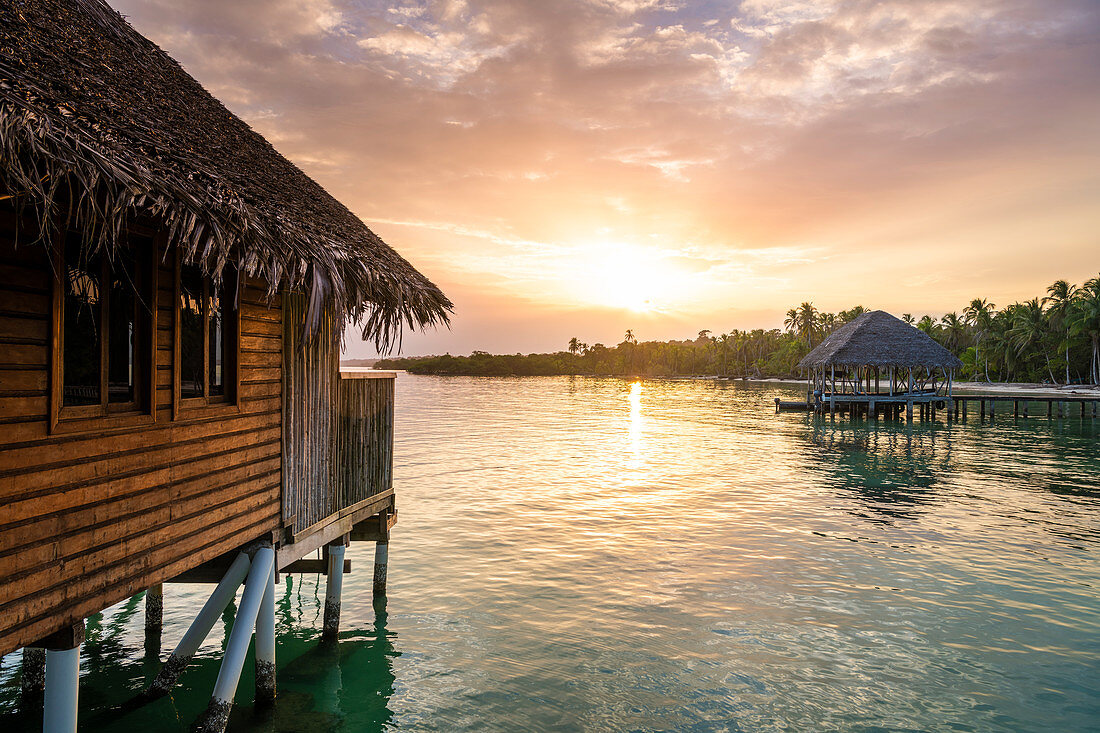This photograph captures a serene tropical island scene during sunset. In the foreground, a wooden hut on stilts extends into the still, bluish waters. The hut, featuring brown wood slat siding and a thatched roof, includes a deck with railing and two windows, hinting at simple yet charming accommodations. Adjacent to the main hut is an open-sided structure, possibly a boat dock, with a small boat tied up, equipped with a trolley motor. The backdrop reveals a white sandy beach lined with tall palm trees, emphasizing the tropical setting. The sky, heavy with grey clouds, is painted with the warm hues of the setting sun, reflecting beautifully upon the water's surface. The scene is void of human presence, allowing the natural beauty and tranquility of the locale to dominate.